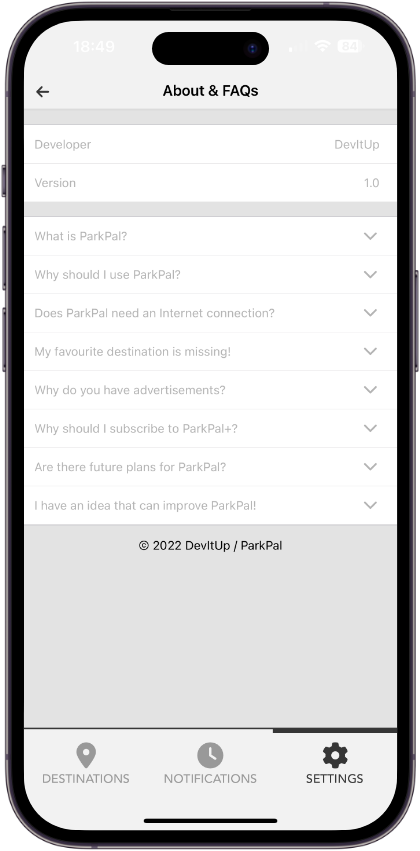This detailed illustration depicts a smartphone displaying the user interface of an app called "Park Pal." The smartphone frame has a very dark gray color, highlighting the screen's realistic appearance. The top border of the screen features a light gray background with white text showing the time as 18:49. On the right side of this border, there are icons for the battery and Wi-Fi signals. The phone also includes a notch— a black rectangle with rounded corners—at the top center.

Beneath the notch, in bold black font, the screen prominently displays the text "About and FAQs." The main background here is white, contrasted with very light gray text for the content, which might be a bit difficult to read. On the left side, headings such as "Developer" and "Version" are listed above a gray divider line that extends from left to right.

Below the divider, bold text asks several questions about the app: "What is Park Pal?" "Why should I use Park Pal?" "Does Park Pal need an internet connection?" and "My favorite destination is missing." Each question has an inverted triangle to the right, indicating a dropdown menu for users to click and reveal answers.

Further questions include: "Why do you have advertisements?" "Why should I subscribe to Park Pal Plus?" (denoted by a plus sign), "Are there future plans for Park Pal?" and "I have an idea that can improve Park Pal."

At the bottom, the background shifts back to light gray. Here, the copyright symbol followed by "2022 Develop Up/ Park Pal" is displayed. Another footer area at the very bottom of the screen shows three sections: "Destinations" on the left, "Notifications" in the middle, and "Settings" on the right, all in gray font.